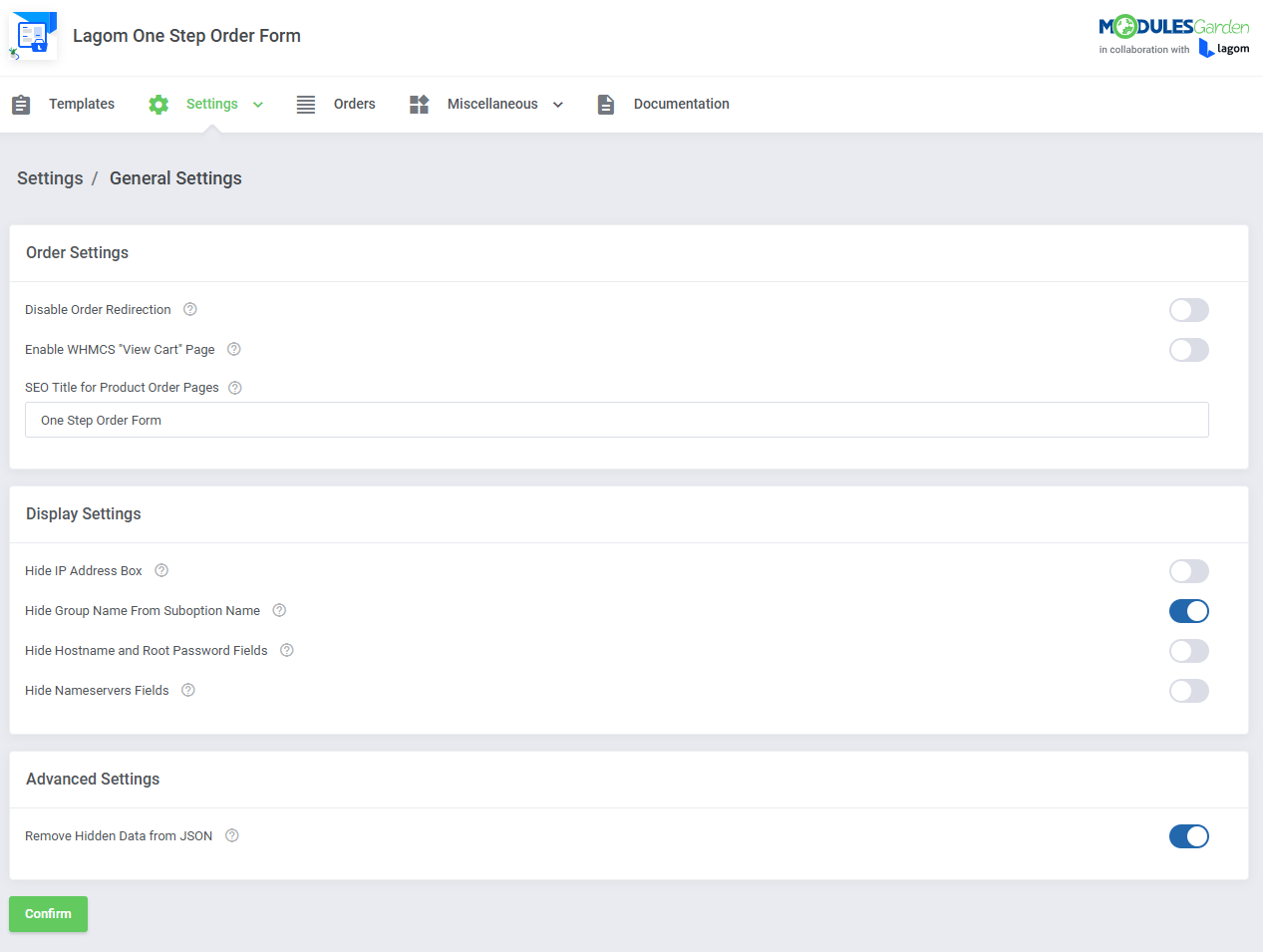This image is a detailed screenshot of a digital order form interface, specifically for the "LAGOM One Step Order Form." 

#### Top Left Section:
- **Icon & Title**: A square icon is positioned to the left, followed by the text "LAGOM One Step Order Form," clearly spelled out as L-A-G-O-M.

#### Top Right Section:
- **Modules Garden Logo**: On the top right, the logo for "Modules Garden" is prominently displayed.

#### Left Sidebar:
- **Options List**: Below the logo, a vertical menu features various categories: Options, Templates, Settings, Orders, Miscellaneous, and Documentation. The "Settings" category is selected, highlighted in green, while the rest remain in grey.

#### Main Content Area:
- **Settings Tab**: The main content area has a grey background indicating the active "Settings" tab.
  - **General Settings**: At the top left of this tab, "General Settings" text is prominently displayed.
  - **Disable Redirection**: A labeled section near the top left includes a small question mark icon for more information. 
  - **Hide Group Name from Suboption Name**: Toward the far right, a toggle switch is turned on for this setting.
  - **Browser's Title Bar**: Below this section, a text box is allocated for customization.
  - **Hide VAT Number Field 4**: Includes a dropdown menu with no selection made.
  - **Hide IP Address Bar**: Accompanied by an off toggle switch.
  - **Hide Host Name and Root Password Fields**: Another section with an off toggle switch.
  - **Hide Name Servers Fields**: Includes a toggle switch that is also turned off.
  - **Remove Hidden Cells from JSON**: A toggle switch is turned on for this option.

#### Bottom Left:
- **Confirm Button**: A green button labeled "Confirm" is clearly visible at the bottom left.

The meticulous layout, with specific toggles and settings options, ensures a user-friendly experience for managing order forms.